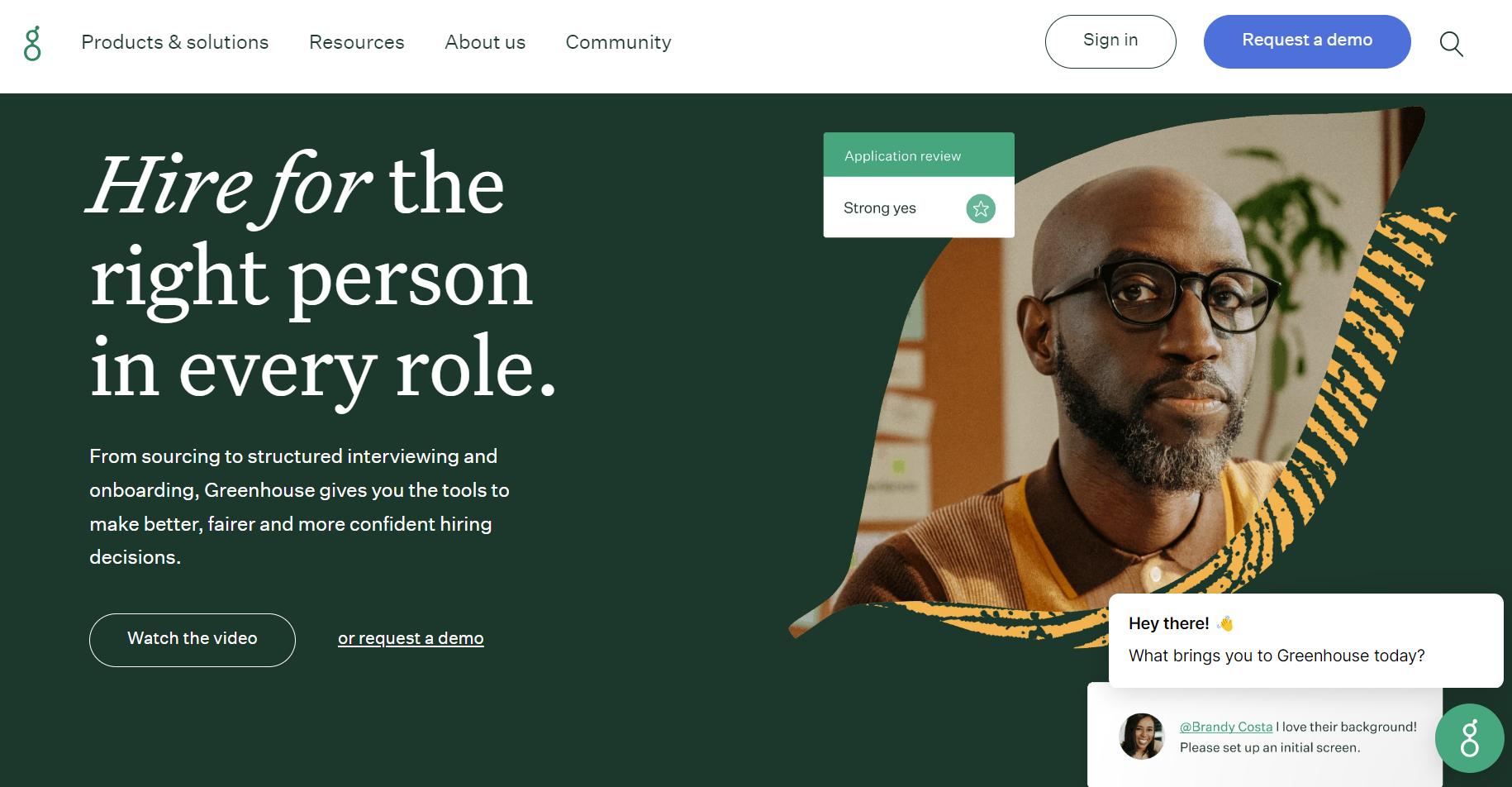Website Screenshot Description:

The image showcases a landscape-oriented screenshot of a website without defined outer borders. At the top, there's a horizontal white header featuring a green 'G'-shaped icon on the left. Adjacent to the icon, various clickable options are listed in grayish-black font, including "Products & Solutions," "Resources," "About Us," and "Community." On the top right, there's an oval-shaped sign-in button with a white background, gray border, and gray text. Next to it, a longer blue oval button with white text reads "Request a Demo."

Below the header, a long green rectangular banner spans the width of the page. On the left side of this banner, white text states, "Hire for the right person in every role." Beneath that, subtext reads, "From sourcing to structured interviewing and onboarding, Greenhouse gives you the tools to make better, fairer, and more confident hiring decisions." A white-bordered text bubble within the banner, also featuring white text on a green background, prompts users to "Watch the Video," followed by a white link that says "Or Request a Demo."

To the right of this banner, there's an application review box. The top portion of this box is green with white text, and beneath it, a long white box displays the phrase "Strong Yes" alongside a star icon.